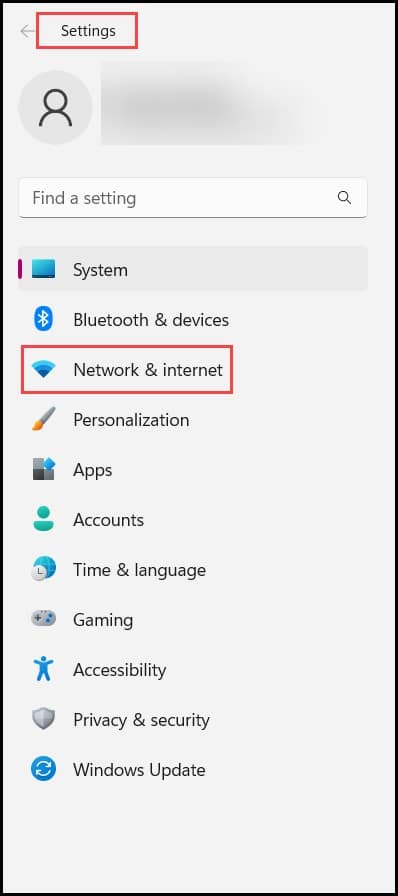The image is a screenshot of the 'Settings' menu in a Windows environment. The settings menu is displayed within a grey box bordered by a black outline. At the very top, the title "Settings" is prominently displayed, encircled by a red rectangle to highlight it. Directly below is a circular user profile icon featuring a generic person image, indicating that no custom profile picture has been uploaded. The username is presented in grey text, showing it is not actively selected or editable at this moment.

Beneath the profile icon is a white search bar with a magnifying glass icon, labeled "Find a setting," where users can type to search for specific settings. Following the search bar, a vertical list of various settings categories is presented. These categories include:

1. System
2. Bluetooth & Devices
3. Network & Internet
4. Personalization
5. Apps
6. Accounts
7. Time & Language
8. Gaming
9. Accessibility
10. Privacy & Security
11. Windows Update

Each category is represented by its respective icon to the left. Most icons are blue, except for the Personalization icon, which has a hint of yellow. The category "Network & Internet" is highlighted with a red rectangle around it, indicating this is the current selection or the active page within the settings menu.